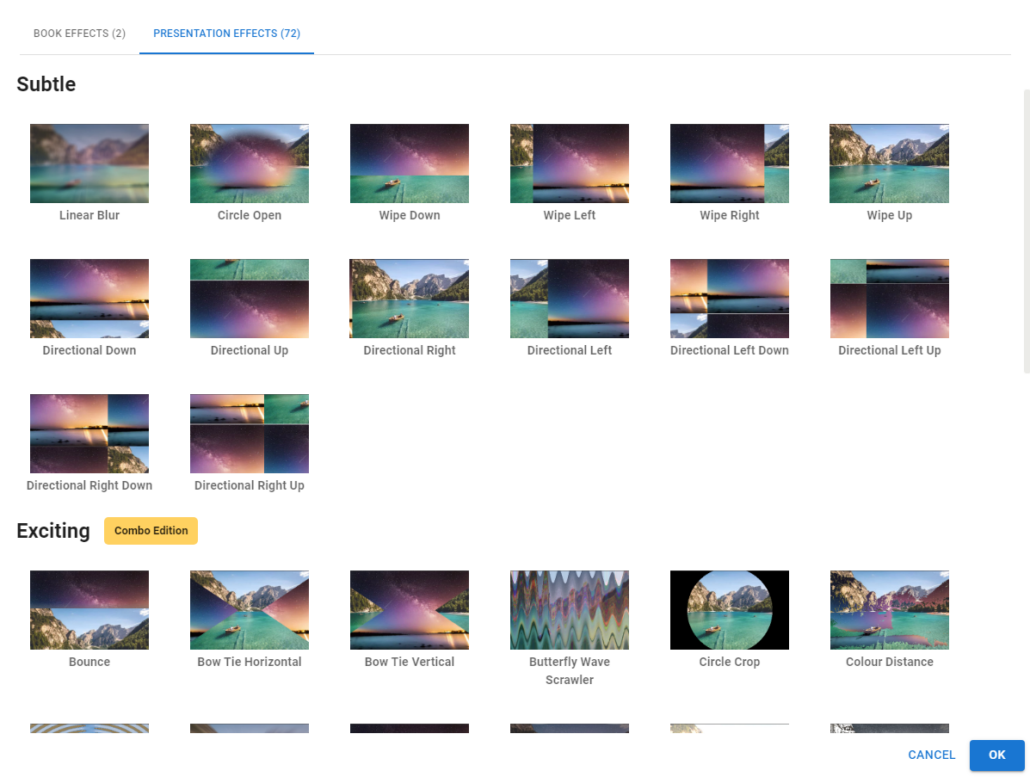This image is a screenshot from a webpage showcasing a gallery of photo effects. The background of the webpage is predominantly white, with the upper left-hand corner featuring a gray-colored section. In gray text in the top left, it reads "Book Effects (2)," and to the right of that in blue font, it states "Presentation Effects (72)." The bold black font in the upper left corner says "Subtle."

The gallery is organized into three full rows and a partial row, with each row containing six items. The images in these rows seem to be various filters and overlays applied to the same base photo. This base photo features a serene scene with water stretching from left to right, a mountain range in the background, and a blue sky.

Beneath these rows, there is a section labeled "Exciting," and within this section, there's a gold rectangle with the text "Combo Edition" written in black. This section also displays six different versions of the same base photo, each exhibiting different special effects similar to those in the "Subtle" category.